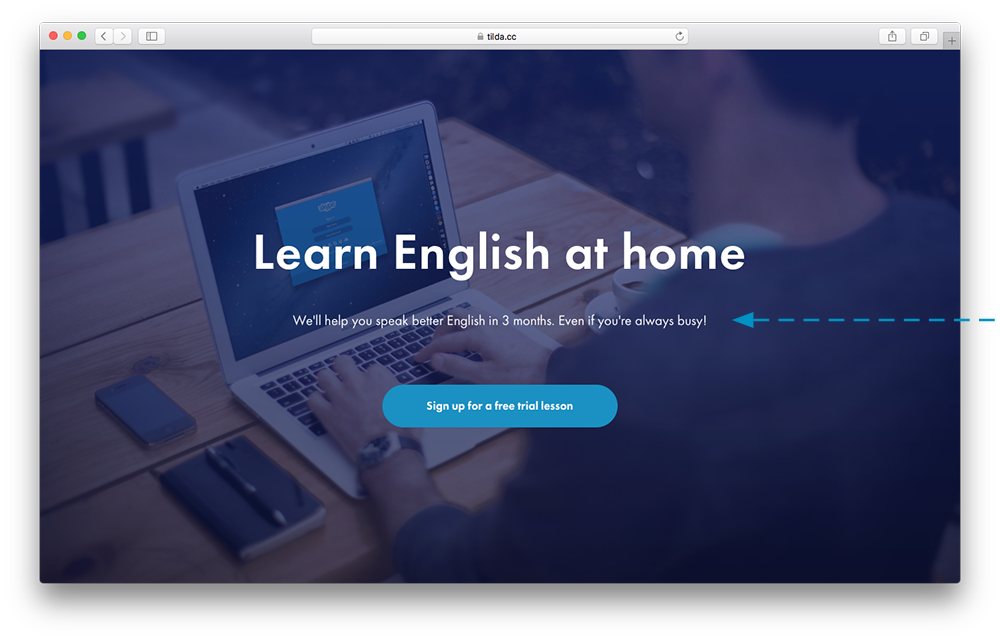In the top left corner of the image, there is a series of colored circles—red, yellow, and green—followed by left and right arrows, a lock icon, and text that reads "tilde.cc". A white address bar is prominently displayed next to a refresh button, a square with an up arrow, and two squares side by side. Central to the image, there is a Macbook laptop with a recognizable old-style design featuring black keys and a silver casing, positioned on a wooden table with a dirt background. The laptop screen shows the Skype application. To the left of the laptop, a smartphone is visible alongside a small Moleskine notebook with a pen resting on top. The person using the laptop is typing, wearing a gray shirt with a white collar, a watch on their left wrist, and has short hair. At the center of the screen, there is a promotional text that reads, "Learn English at home. We’ll help you speak better English in three months, even if you're always busy." Below this text, a blue arrow points to the left and there are dash marks depicted as dash-dot-dot-dot. Additionally, there is a blue circle with the text "Sign up for a free trial lesson." This image portrays a website for learning English at home, displayed on a Mac browser with the URL "tilde.cc".